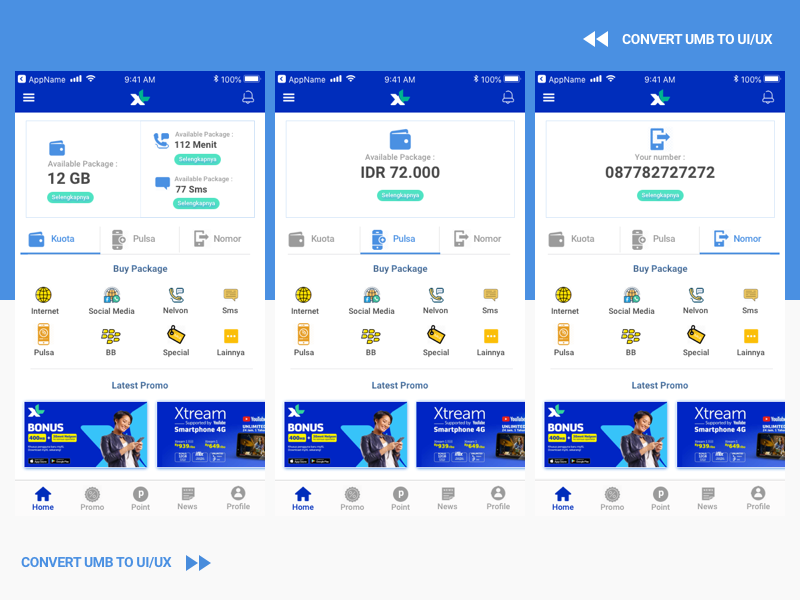Here is a polished and detailed caption for the image described:

"This converter page displays three distinct phone screenshots in a vertical column, each associated with different details of a telecommunications app. In the first screenshot, captured at 9:14 AM, the app displays available packages: 12 GB of data, 112 minutes labeled as 'MENIT', and 77 SMS messages. Options to purchase packages are listed as 'KUOTA', 'PULSA', and 'NOMOR'. Additionally, eight identical icons across all screenshots are labeled as: 'Internet', 'Social Media', 'Nelvon' (the phone company's name, spelled 'N-E-L-V-O-N' beneath a telephone icon), 'SMS', 'Pulsa', 'BBspecial', and 'LAINNYA'. 

The second screenshot mirrors the first, except it indicates a package availability of IDR 72,000 in place of the previous numeric data. The third screenshot is also identical in structure, with the primary difference being the display of a phone number: 0877-827-27272. All three screenshots include identical bottom-row icons for various app features: 'Home', 'Promo', 'Point', 'News', and 'Profile'. 

At the very bottom of the screen, the image displays different advertisement banners such as 'X-Stream', 'Bonus', and additional icons explicitly titled as 'Convert UMV to UI/UX'."